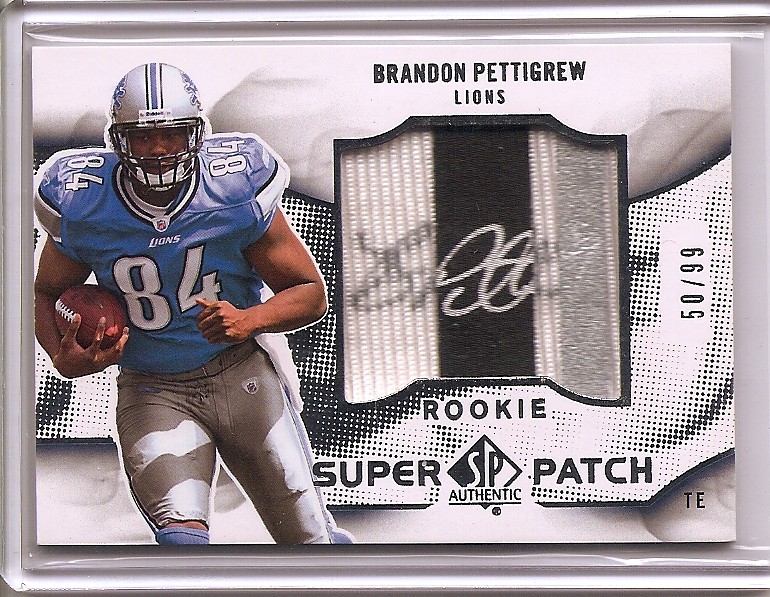This image depicts an NFL football trading card featuring Brandon Pettigrew in a Detroit Lions uniform. The card prominently displays "BRANDON PETTIGREW" in capital letters across the top. A photograph of Pettigrew, wearing a blue Lions jersey with white numbers (84) on the shoulders and chest, occupies the left side. He is seen holding a football in his right hand, wearing a silver helmet with a blue stripe down the middle.

The card includes several other notable details: on the right-hand side, beneath the main text, it says "50/99," indicating its limited-edition status. It also features "Rookie" and "Super Patch," affirming the card’s significance and the authenticity of the patch it contains. Additionally, "TE" for Tight End is printed in the bottom right corner. 

The card is housed in a protective top loader case, with a clear plastic sleeve inside, ensuring its preservation. Although there are some visual complexities in the background, such as a black-and-white photo of arms and what appears to be the image of a door or window, the main focus remains on Brandon Pettigrew in action.